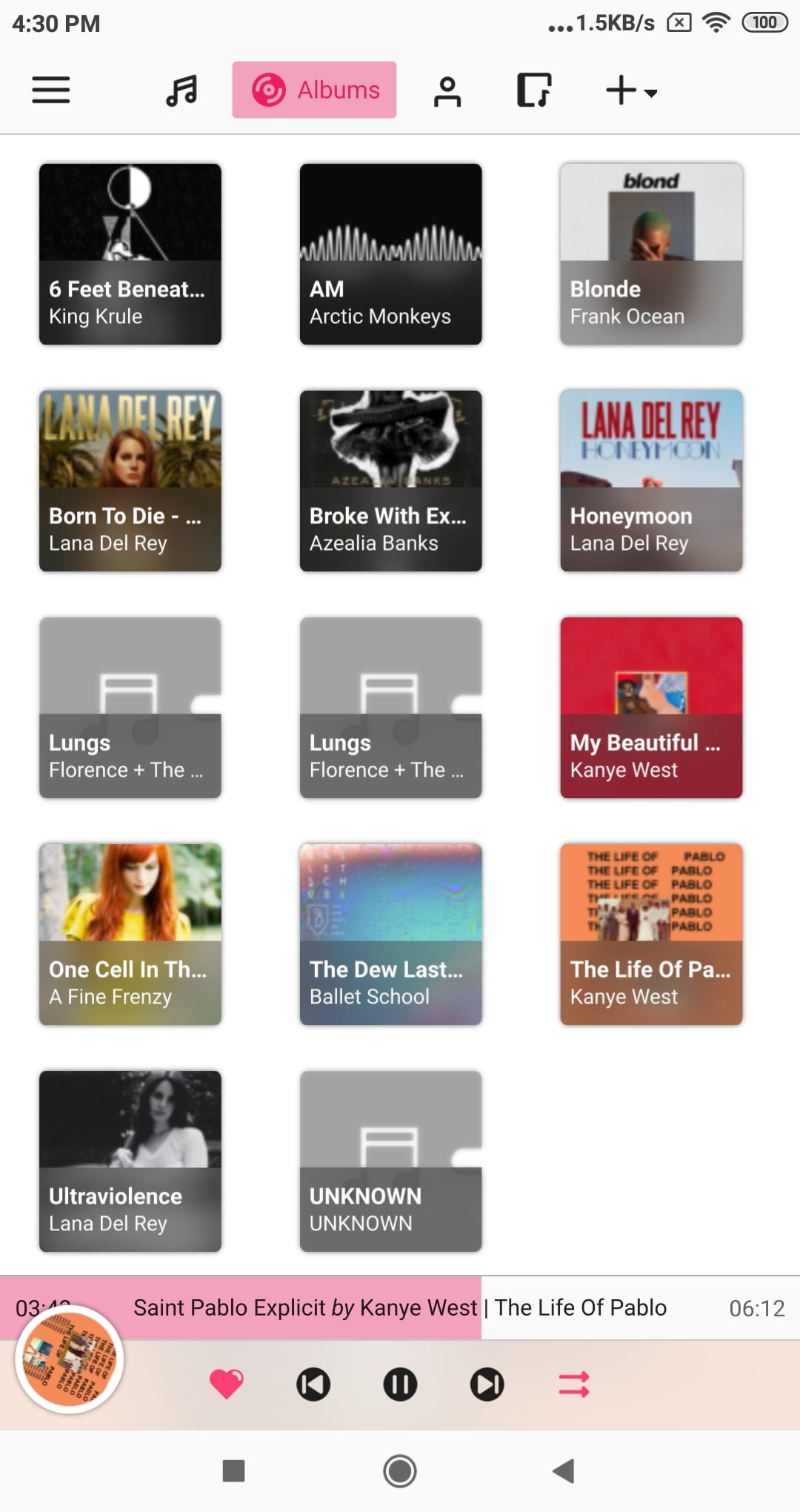A vertically-oriented smartphone screenshot, likely taken from an iPhone or Android device, displaying a music player app. The upper portion of the screen features a thick gray strip containing various status indicators: the time displayed at 4:30 p.m. on the upper left, and the upper right showing three black dots, a 1.5 KB/s data indicator, Wi-Fi signal strength, and 100% battery life.

Below the time, there are three horizontal lines and several icons: a music note icon, an "albums" section highlighted in pink, a person icon, another music note with a square plus sign, and a list of selectable music albums. The listed albums include:

- "Six Feet Beneath"
- "A.M." by Arctic Monkeys
- "Blonde" by Frank Ocean
- "Born to Die," "Born With"
- "X..."
- "Honeymoon" by Lana Del Rey
- "Lungs"
- "Other Lungs"
- "My Beautiful" by Kanye West
- "One Cell in the Sea"
- "Fi-Fi and Frenzy"
- "The Do Last" by Ballet School
- "The Life of..." (truncated)
- "PA..." by Kanye West
- "Ultra Violence" by Lana Del Rey
- "Unknown"

At the bottom of the screen, the currently selected track is "St. Pablo (Explicit)" by Kanye West from the album "The Life of Pablo," with a duration of 6 minutes and 12 seconds. The control panel includes icons for heart (like), fast forward, rewind, pause, and play functions. There is also a circular user icon visible.